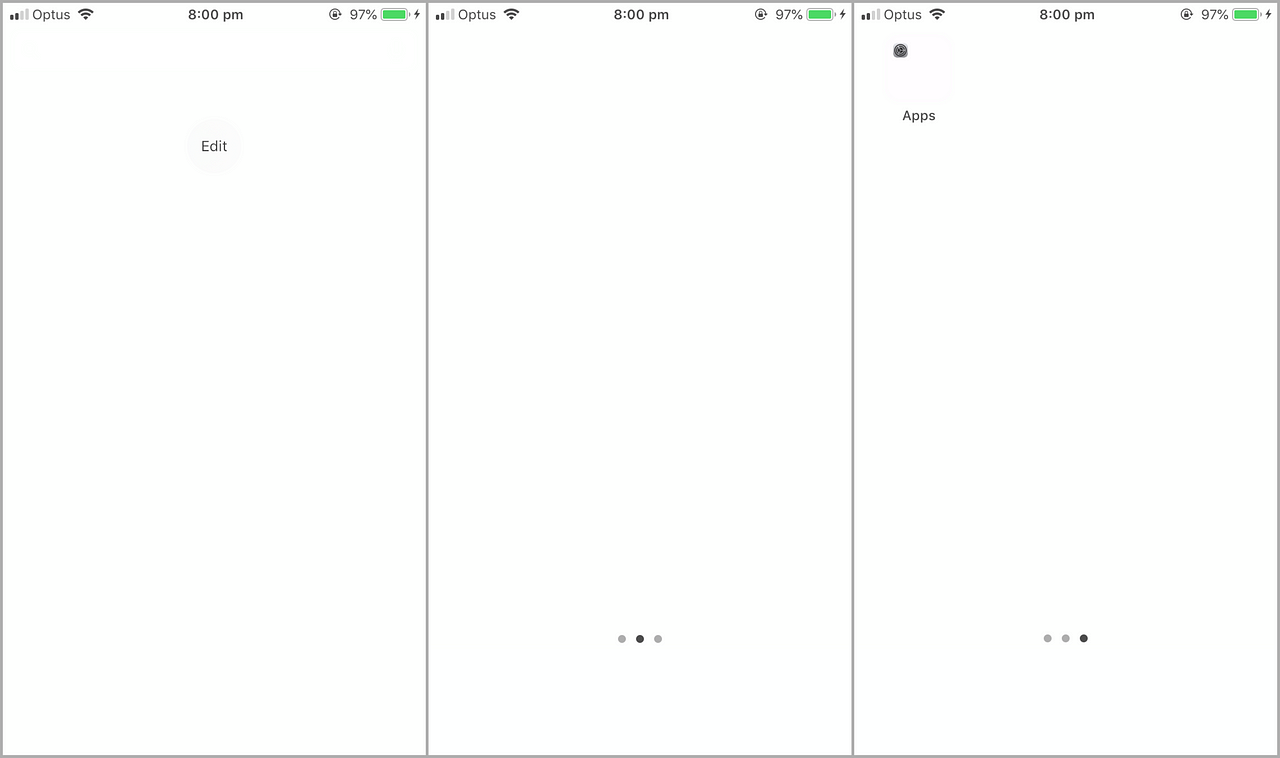The image consists of three sequential screenshots captured at 8:00 p.m., with each screen showing a battery level of 97% and a thunderbolt icon indicating the device is charging.

In the first screenshot, there is a very light gray circle at the center with the word "Edit" displayed inside it.

The second screenshot, appears to be blank except for three navigation dots at the bottom of the screen. The second dot is black, signifying it as the active screen, while the other two are gray.

The third screenshot features a small gray square labeled "Apps". Behind this small black square, there is a very light beige square. Similar to the second screenshot, this screen also has three navigation dots at the bottom, but this time, the third dot is black, indicating it as the currently active screen.